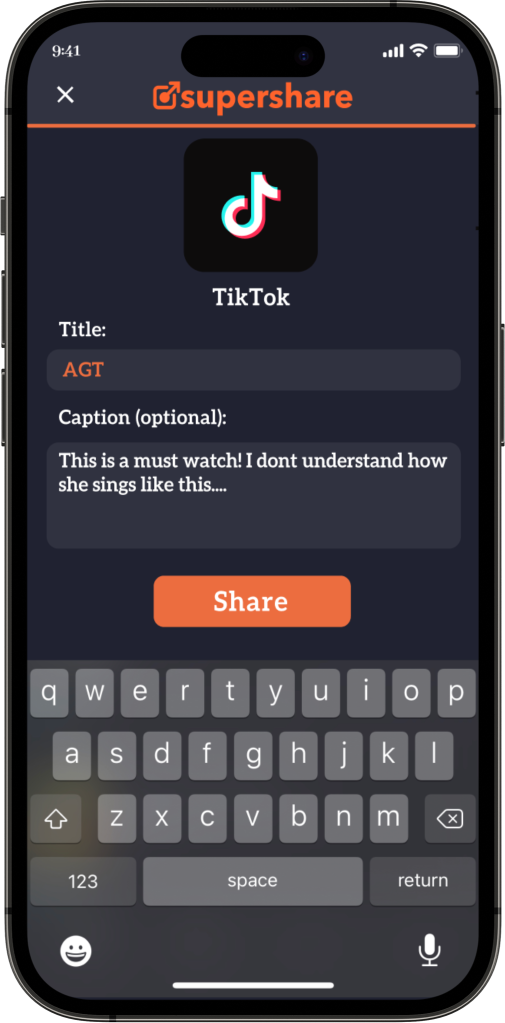The image appears to be a detailed screenshot of an Apple mobile device, encompassing not just the screen content but the physical structure of the device itself. The phone has curved edges, and on the right side, approximately midway up, a prominent main button is visible. On the upper left side of the device, the volume up button is present, and just above it, a smaller lock button can be seen.

The majority of the screen is black. In the upper left corner, the current time is displayed, while the upper right corner shows icons for cellular signal strength, Wi-Fi strength, and battery level.

At the top portion of the screen, there is a section highlighted in red or orange with the text "SuperShare" accompanied by a small icon on its left and a thin orange line below. Underneath this header, the TikTok icon followed by the word "TikTok" is visible. Moving further down, there is a label "title:" to the left, with the text "AGT" in orange beneath it. Below this, in white text, it states "Caption, optional:". The caption reads, "This is a must watch. I don’t understand how she sings like this....".

Following the caption is an orange button with white text labeled "Share". At the very bottom of the screen, the standard mobile device keyboard is displayed, complete with all the letter keys. On the bottom left of the keyboard, there is an emoji icon, and on the bottom right, a microphone icon is visible, indicating the option to record audio.